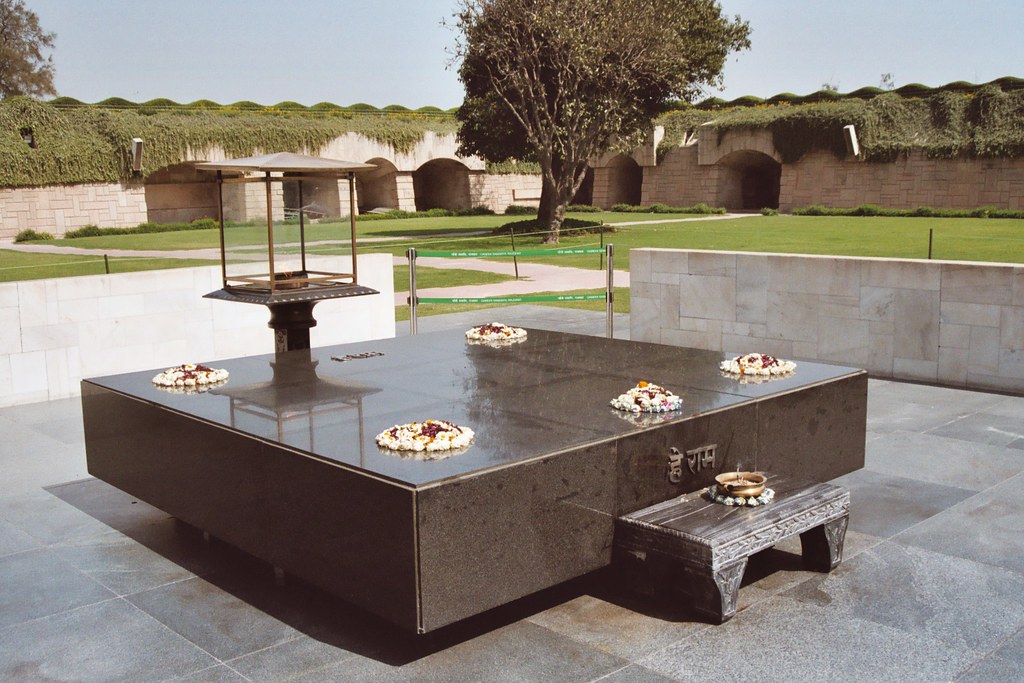The image captures a picturesque courtyard framed by a mix of old and new elements. In the center of this serene scene is a large, solid stone table with a polished, reflective top, glistening in the daylight. Placed meticulously at each corner of the table are multiple white, fluffy dessert items, each adorned with vibrant red bits of fruit in their centers. A similar dessert item is positioned in the front, adding to the table's inviting display.

In the immediate foreground, a small dark gray bench supports a bowl, hinting at a tranquil moment of contemplation or offering. The ground beneath is laid with light gray square tiles, contrasting the outdoor setting with an air of refined elegance. To the left, a light gray wall rises, while the right side showcases a darker gray wall adorned with green blockades and supported by two poles.

Further back, the courtyard extends into a meticulously maintained lawn, featuring a lone large tree with dark green leaves, providing a touch of nature's majesty. The backdrop reveals fortified stone walls, possibly remnants of an ancient fort, now softened by ivy and vines. Embedded within these historical walls are modern speakers, blending seamlessly with the past. The blue sky overhead completes this harmonious blend of nature, history, and modernity, encapsulating the essence of a fancy Asian garden or park.